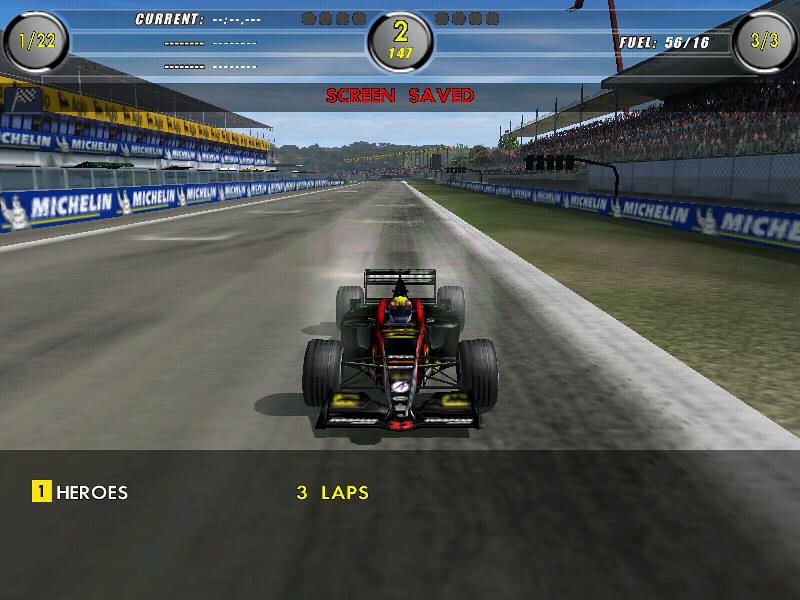In this vibrant scene, an asphalt surface, likely a racetrack, features prominently. To the right, a crisp white line demarcates the boundary followed by a strip of lush green. Further to the extreme right, a large Michelín banner in bold white text, accompanied by the iconic Michelín Man, stands out against the backdrop. 

Beyond this, a stone wall ascends towards stands where enthusiastic fans are seated under a protective canopy, shielding them from the sun. The sky overhead is a clear, vivid blue. 

On the left side, another Michelín banner is visible against a blue wall with white text. Below this, a yellow element stands out, marked with "screen saved" at the top. In the top left corner of this element is a large circle, yellow inside, containing the numbers 1 and 22, with various dots and numbers such as 2, 1, 7, and 16/3. The right side of this display reads "fuel," adding to the rich tapestry of the scene.